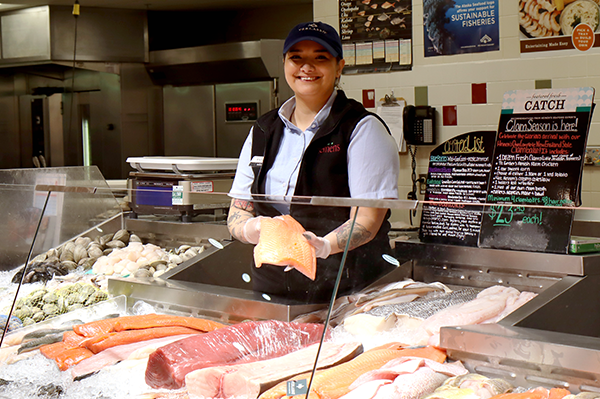In the bustling setting of a seafood market within a grocery store, a smiling white woman stands proudly behind the fish counter. She wears a distinctive red vest emblazoned with the name of her workplace, though the exact words are hard to make out. Her attire includes a black baseball cap and white gloves, while her hair is neatly tied back in a ponytail. She showcases a piece of raw fish, likely salmon, amidst a vibrant display of various seafood including fish, clams, and shellfish, all arranged within a glass display case designed to keep the products fresh and uncontaminated.

Her arms, adorned with tattoos, can be seen as she holds the fish confidently, indicating her comfort and experience in this environment. Behind her, industrial-sized refrigerators and a digital scale are visible, reinforcing the market’s professional setup. The background is busy with posters and sandwich boards announcing seasonal specials, prominently featuring the phrases "Catch" and "Clam season is here." The overall ambiance reflects a well-organized and dynamic seafood section, where quality and freshness are at the forefront.